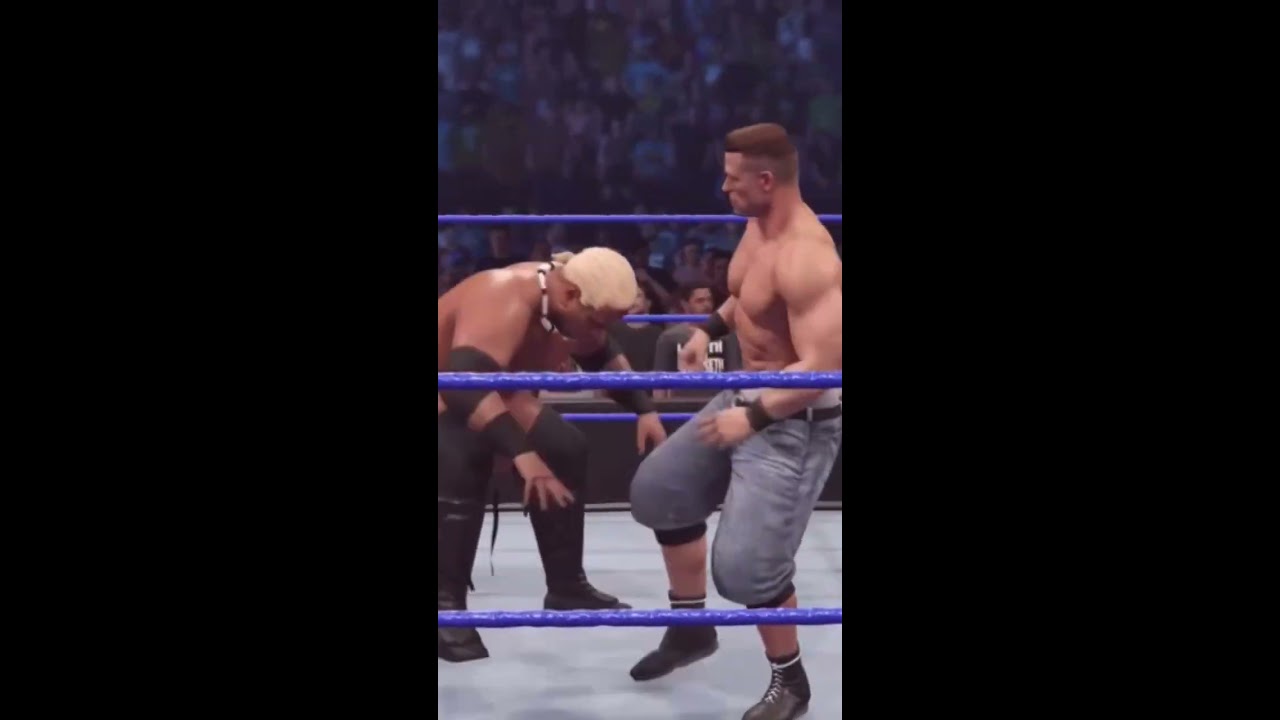In this highly detailed image, we see a realistic depiction of a wrestling match, likely from a video game. The wrestling ring features deep blue ropes on all sides and a light blue mat. In the background, there's a large, somewhat blurred audience, separated from the action by a black barrier. 

On the right-hand side stands John Cena, muscular and shirtless, wearing light blue jean shorts that extend to his knees. He has black knee pads, black boots, and black wristbands. His short brown hair is shaved on the sides, and he appears to be engaging with his opponent.

Opposite him is Samoa Joe, who appears hunched over. He sports bleached blonde hair tied in a back ponytail, a puka shell necklace, black elbow pads, and black wrist tape. His attire includes full-length leather pants, black knee pads that extend to black boots with kick pads.

The overall scene captures the intense moment of confrontation between the two wrestlers, set against the vibrant backdrop of a captivated audience.